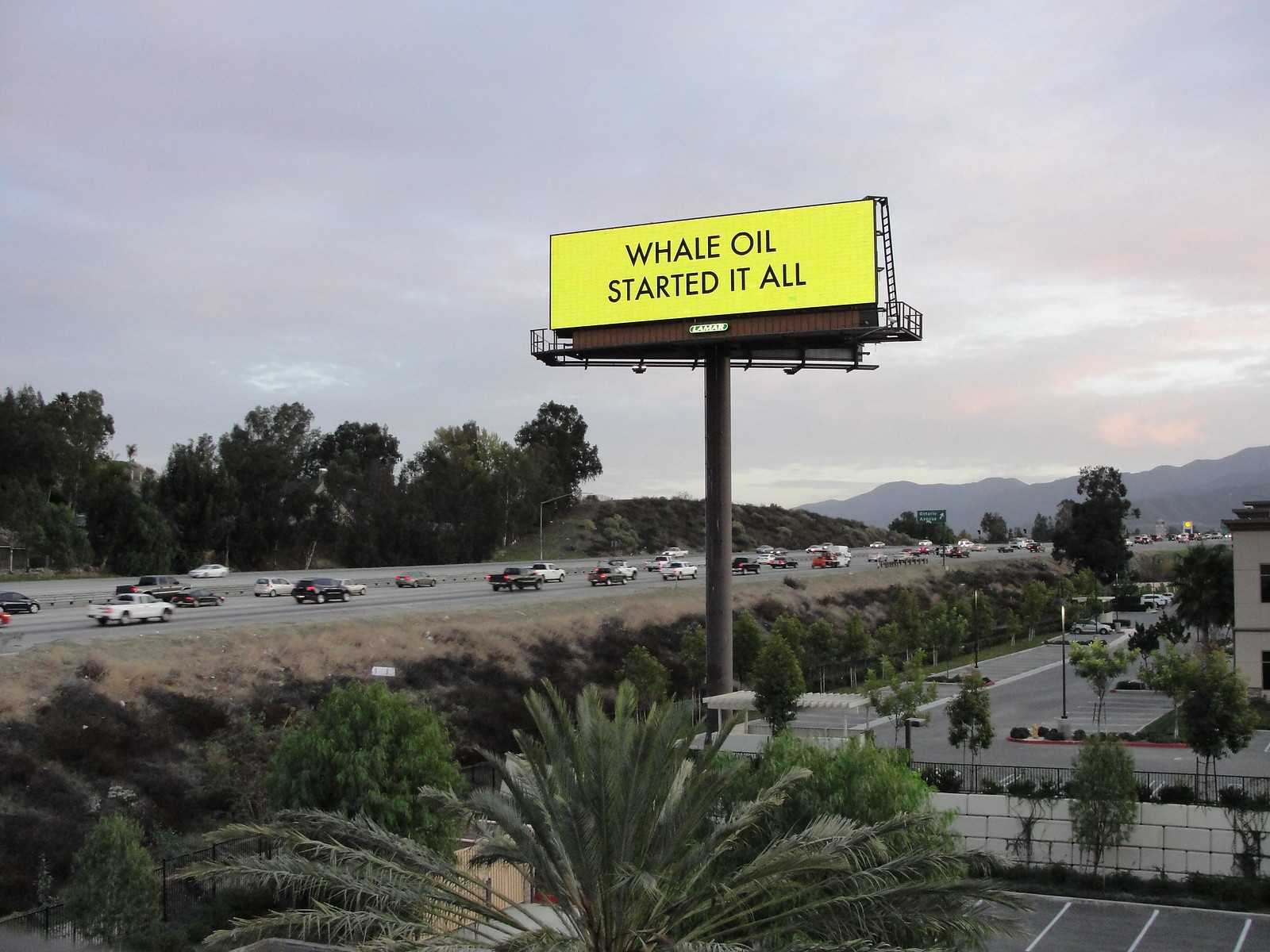The image depicts a color photograph taken from a high vantage point, showcasing a multi-lane interstate highway with substantial traffic, including white, black, and red cars moving in both directions. Centrally positioned is a tall billboard on a high brown post, prominently featuring a yellow background with black block letters that read "Whale Oil Started It All," accompanied by a small Lamar Company logo below. Surrounding the highway is a lush tropical landscape with green trees and plants, a large bush-like tree in the foreground, and a low hill. On the right-hand side of the image lies a mostly empty parking lot adjacent to a small office building. In the distant background, a range of tall mountains stretches under a cloudy, hazy blue sky.